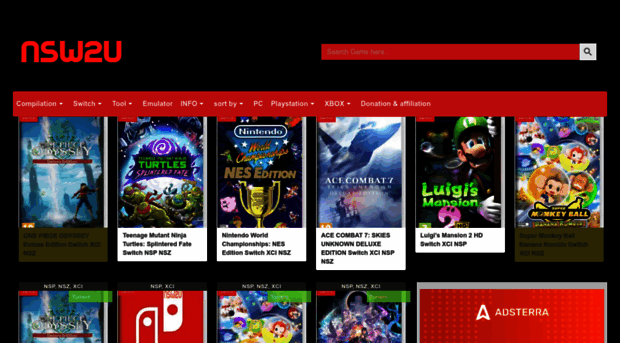The image shows a "NSW2U News" webpage set against a predominantly black background, with a red section in the upper left corner. At the top, there's a red search bar with "Search games here" written in white, accompanied by a white button featuring a black magnifying glass icon.

Below the search bar, several red navigation tabs are aligned horizontally, each featuring a pull-down menu: "Compilation," "Tools," "Emulator Info," "Sort By," "PC," "PlayStation," "Xbox," and "Donation and Affiliation."

The main content area is filled with rows of game or film titles. Some of the visible titles include "Showtime," "Contra," "Tomb Raider," "Mario," "Juju Kaisen: Cursed," and "Hitman." The page appears to offer a mix of game and film-related content, though the exact nature of some titles is unclear.